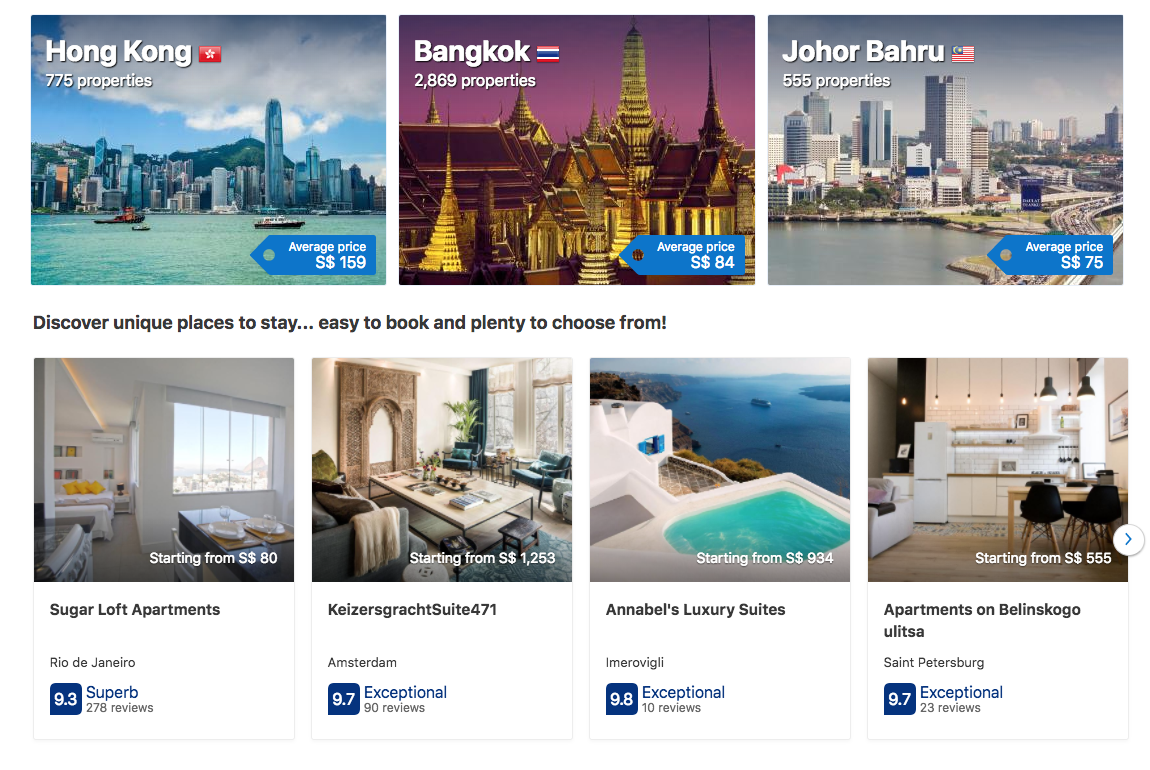This image appears to be taken from a travel website, showcasing a selection of destinations in a structured layout. There are two rows, with the top row featuring three blocks, each depicting a different city along with property information.

- **Left Block (Hong Kong)**: The left block presents an image of Hong Kong, indicating that there are 775 properties available. Towards the bottom right corner of the block, there is a small ribbon displaying the average price of properties, which is $159. The image within the block shows a waterfront scene with buildings in the background, suggestive of Hong Kong's iconic skyline.

- **Middle Block (Bangkok)**: The middle block highlights Bangkok, featuring 2,869 properties. Similar to the previous block, a blue ribbon at the bottom right corner states that the average price is $84. The image likely depicts a significant landmark or urban scenery representative of Bangkok.

- **Right Block (Johor Bahru)**: The right block is labeled Johor Bahru and lists 555 properties. The average price, shown on the ribbon in the bottom right corner, is $75. The image associated with this block would typically feature a notable view or landmark from Johor Bahru.

Overall, the layout is clean and organized, with each block providing essential information about the available properties in these prominent travel destinations.